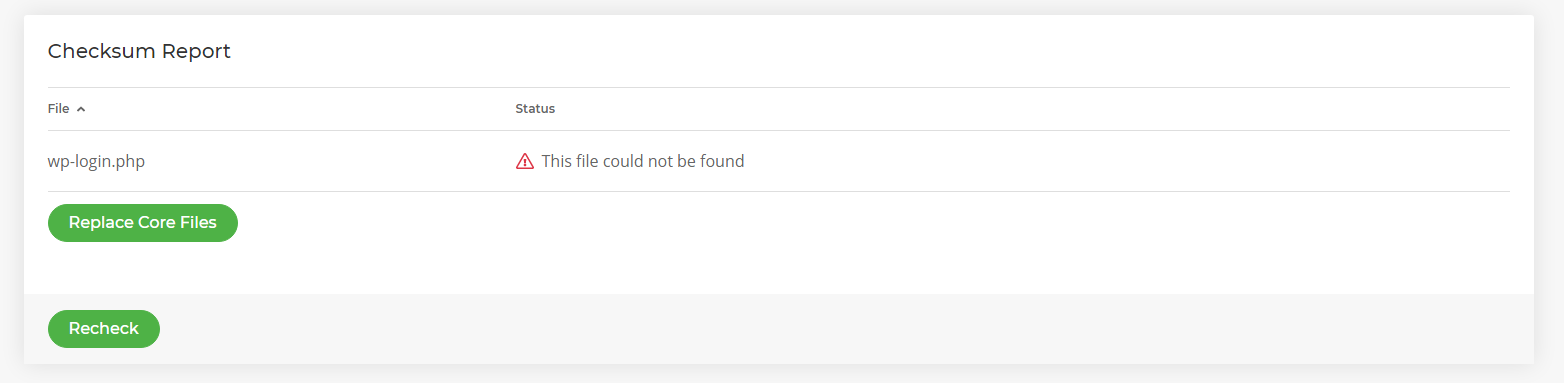This image appears to be a screenshot of a website viewed on a laptop or desktop computer. The webpage background is predominantly white. At the top of the page, there is a small, thin, black font text that reads "Checksum Report." 

Directly below this text is a very thin, almost gray, horizontal line that runs from the left to the right side of the screen. Underneath the line on the left-hand side, there is a smaller black font text that says "File." Beside "File," there is an upward-pointing arrow indicating a drop-down menu.

Beneath this, another thin line separates the sections. Below the line, there is the text "wp/login.php" indicating a specific file path. 

On the right-hand side of this section, there is a significant amount of white space. To the far right, the word "Status" is displayed in small, black font. Underneath "Status," there is a red triangle icon with an exclamation mark inside it, indicating a warning or danger. Next to the red triangle, a gray font message reads, "This file could not be found."

Further down, another thin line is present. On the left side of this section, there is a green cylindrical button with the text "Replace Core Files" written in white. Below this button, with some spacing in between, there is a smaller green cylindrical button with the text "Recheck" also written in white.

Overall, the layout presents a clean, organized design with clear indications for actions related to file management on the website.